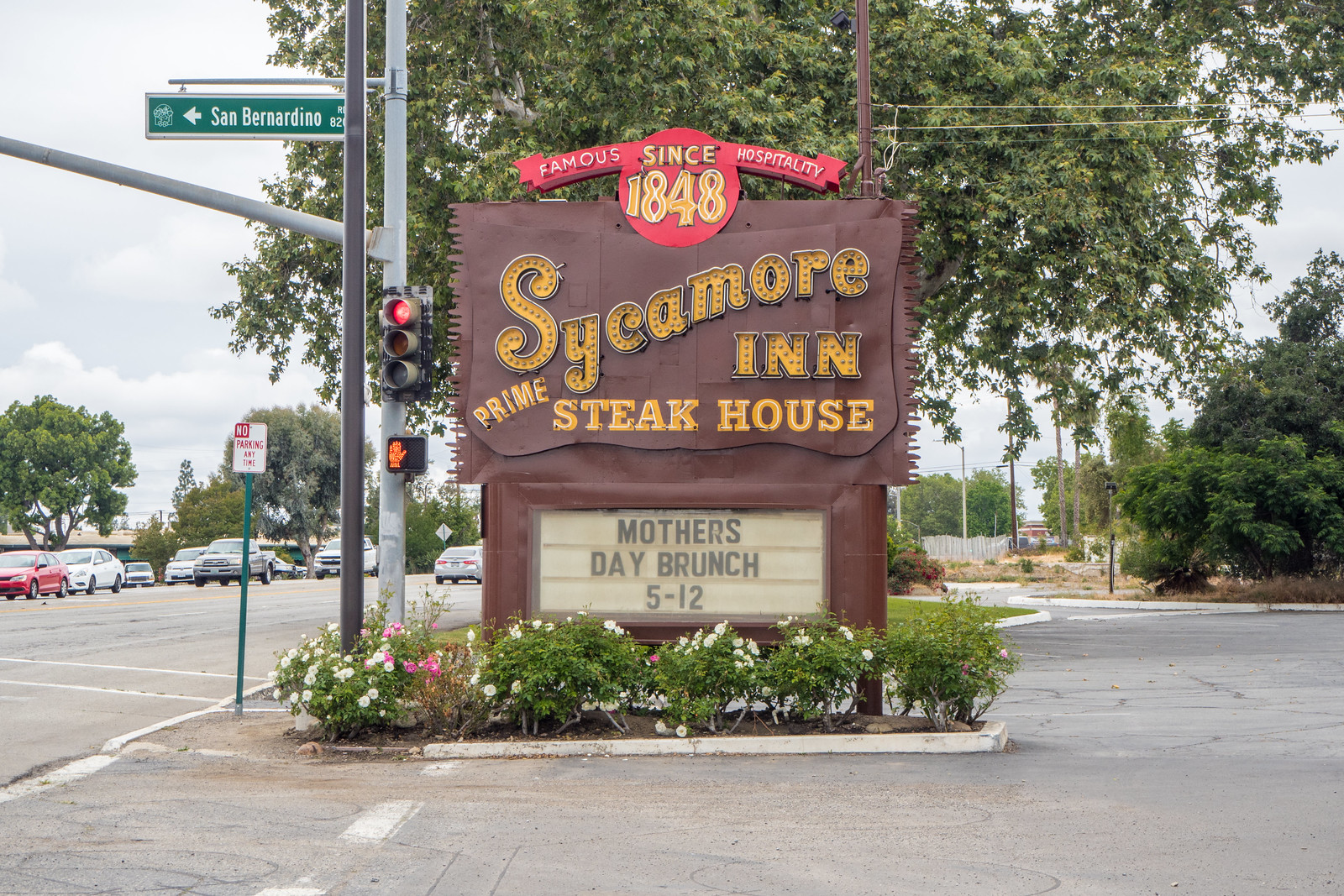The image captures a detailed outdoor scene of a large, stylized brown roadside sign advertising the Sycamore Inn Prime Steakhouse, renowned for its hospitality since 1848. The sign, designed to resemble the side of a log cabin, features a prominent red circle and banner at the top with the phrase "Famous Hospitality Since 1848" in white letters. Below this, "Sycamore Inn Prime Steaks" is displayed in illuminated yellow letters. A white rectangular marquee below the main sign announces "Mother's Day Brunch 5 to 12" in black letters.

The sign is situated in a small curved planter area surrounded by bushes and pink and white flowers. It is positioned near a busy intersection, marked by a tall silver traffic light pole with a green street sign reading "San Bernardino." The traffic light is currently red, and the illuminated crosswalk sign displays a red hand indicating 'stop'. Additionally, there's a red and white "No Parking" sign to the left, and a parking lot opens up to the right. Behind the sign and planter, a large tree adds to the picturesque setting. Various colored vehicles, predominantly white and silver, can be seen moving along the road, enhancing the lively atmosphere.